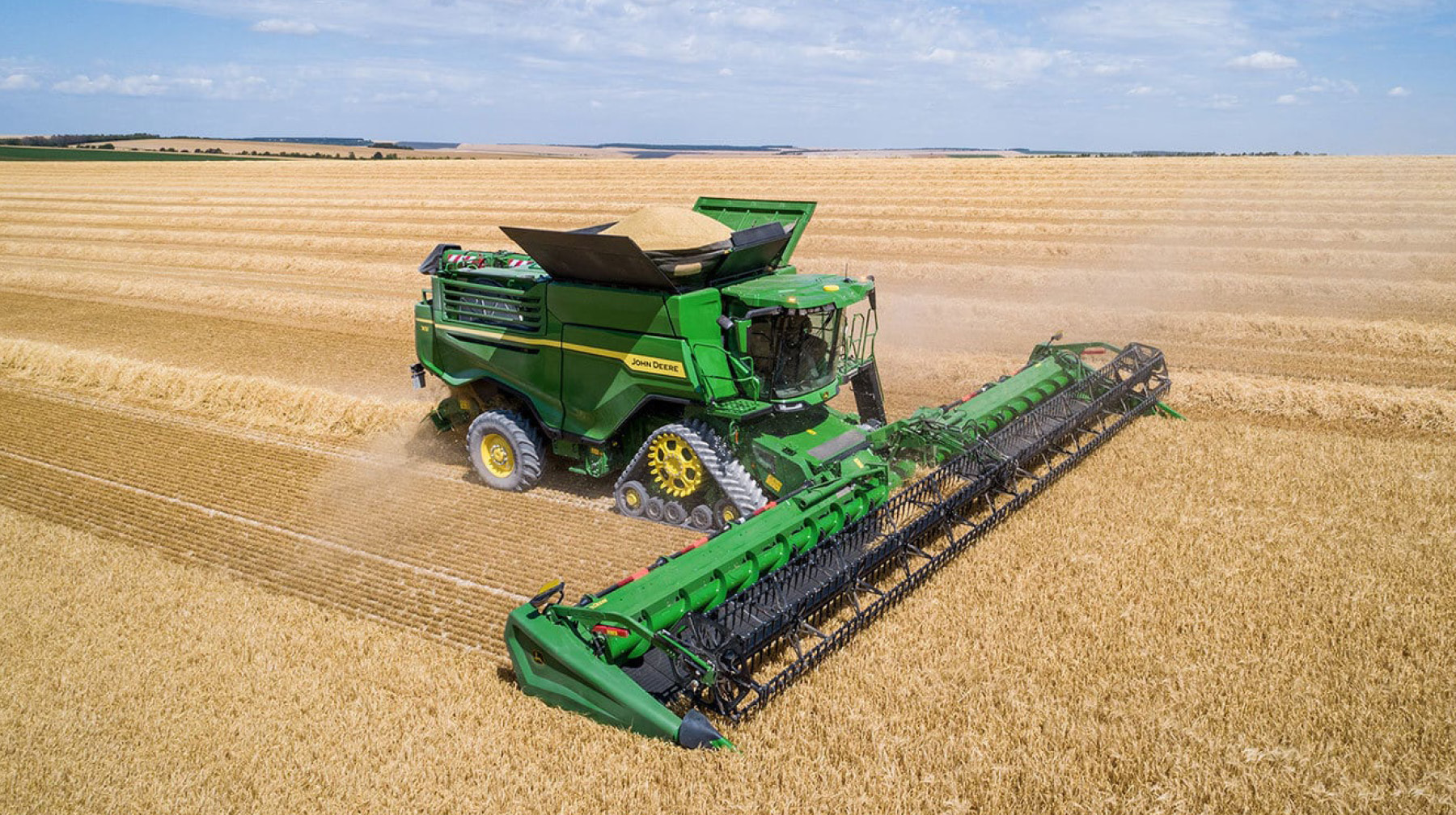This color photo, taken outside during the day, captures an expansive farm scene under a blue sky speckled with white fluffy clouds. The vast, golden grain field, likely wheat, is being harvested by a large, green John Deere combine harvester. The machine prominently features "John Deere" text on its side and is equipped with tank-like tracks in the front and black tires with yellow rims in the rear. In front of the harvester, long blades actively cut through the wheat, separating the seeds from the chaff. The top of the combine has a black container filled with harvested grain, as it moves rightwards across the field, leaving two distinct lines in its wake. In the distant, flat landscape, a slight elevation can be seen, enhancing the vastness of the scene.